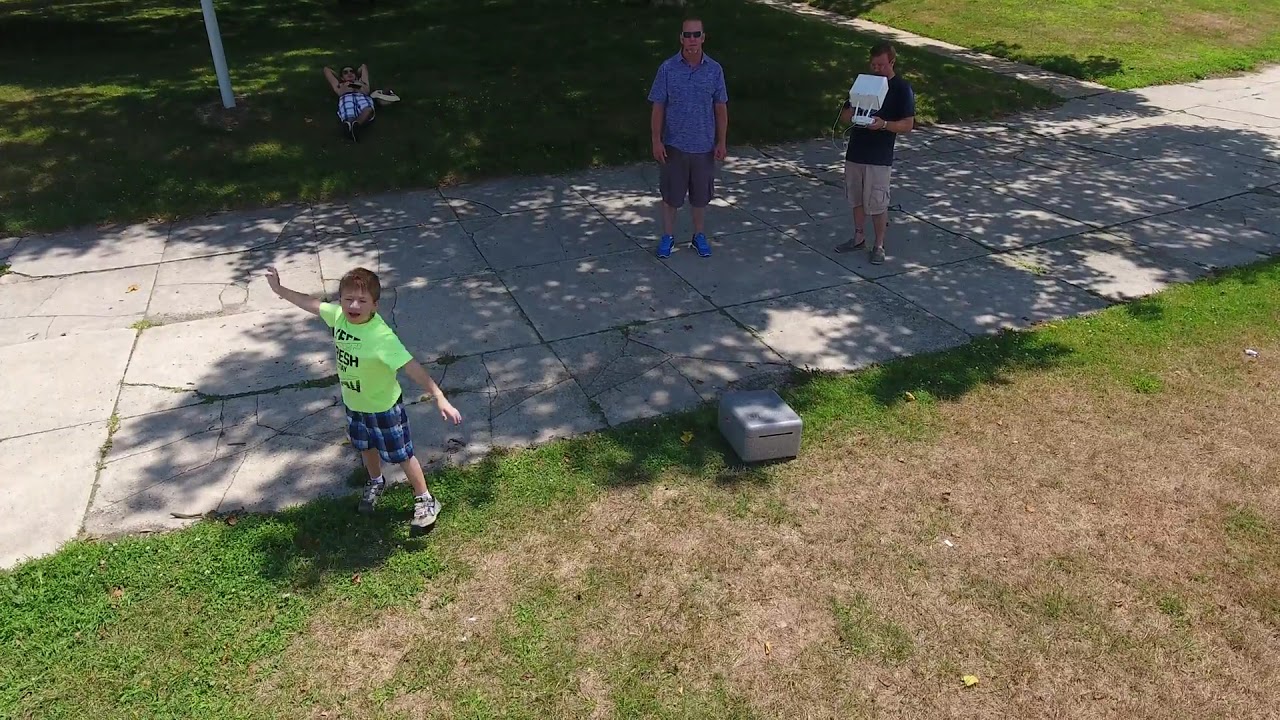In this outdoor photograph, four people are captured in a setting that resembles a park or neighborhood. The scene is centered around a pathway made of large, uneven concrete squares, which runs horizontally across the image. In the foreground on the left, a young boy—approximately ten years old—is posing for the camera with his arms outstretched at shoulder width. He sports a neon yellow t-shirt with some writing on it, paired with blue plaid shorts and white sneakers. His red hair and joyful stance add a dynamic element to the composition. 

To the back and right of the boy, two adult men stand side by side on the pathway. The man on the left wears a blue button-down short-sleeved shirt, gray shorts, and blue running shoes. Next to him, another man holds a white box or possibly a device like a computer screen or controller. This man is dressed in a blue shirt with khaki shorts and brown shoes. Both men seem to be focused on the box, adding an element of intrigue to the scene. 

Further back in the grassy area, a woman is lounging casually with her hands behind her head, donning sunglasses, a beige top, and white and blue plaid shorts. The dry patches of grass transitioning to greener edges frame the pathway and extend the outdoor ambiance. 

Given the slightly elevated angle of the photograph and the presence of a possible controller, it is plausible that this photo was taken using a drone, adding a unique perspective to this seemingly candid family moment.